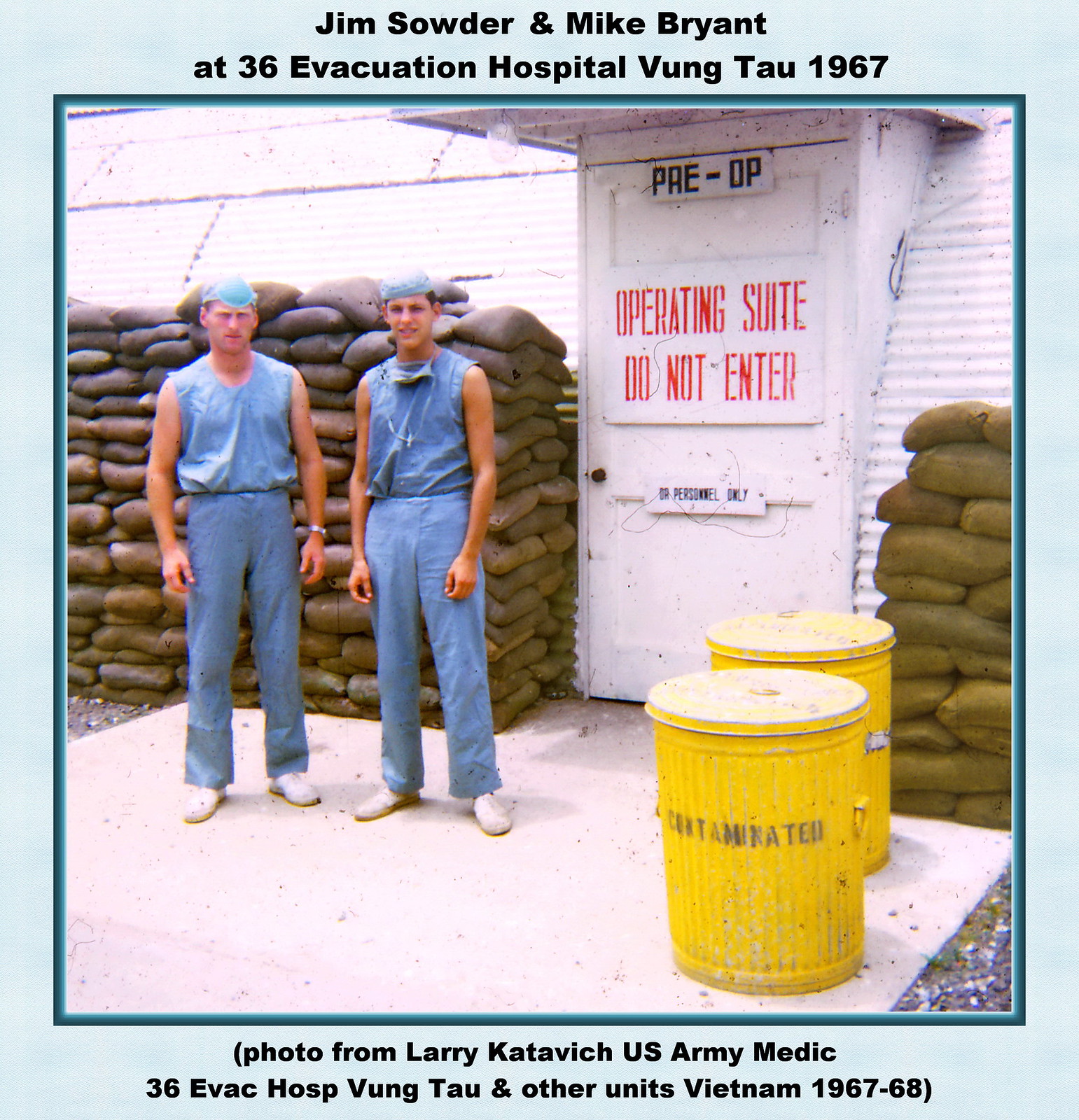The image depicts two young Caucasian men standing outdoors in front of a white sign with black lettering that reads "Operating Suite, Do Not Enter" in red font. They are dressed in blue sleeveless scrubs and blue pants, donning white shoes. The man on the left has a mask on his head, while the man next to him has goggles around his neck and a medical hat on his head. Both appear to be outfitted with personal protective equipment. Behind them and to the right are stacked brown sandbags, reaching about their height. Also visible are two trash barrels, orange in color. One of the barrels has the word "contaminated" written on it in black text. The background of the image features additional white signage and a white ground surface. The top of the image is captioned in black font: "Jim Souter and Mike Bryant at 36 Evacuation Hospital, Vung Tau, 1967." At the bottom of the image, another caption reads in black font: "Photo from Larry Katovich, U.S. Army medic, 36 Evac Hosp, Vung Tau, and other units, Vietnam, 1967-68."